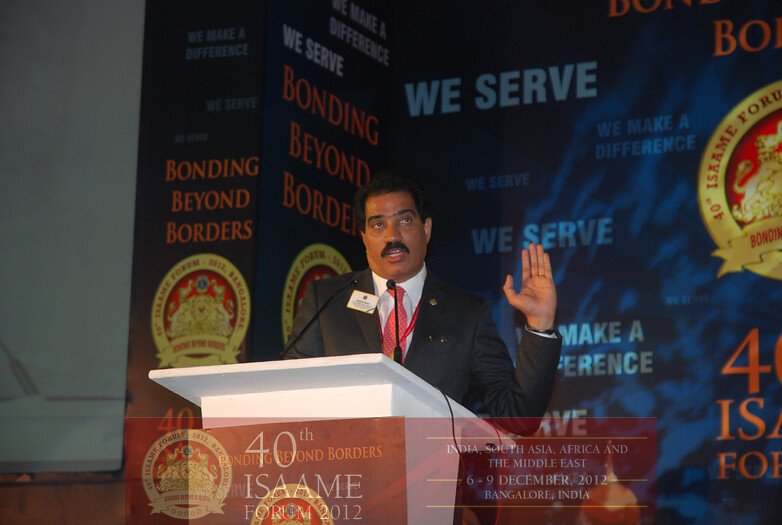In this detailed horizontal rectangular photograph, a South Asian man is making a speech from a white podium, likely at the 40th ISAME Forum held in December 2012 in Bangalore, India. The man, dressed in a dark suit with a red tie and a white shirt, has a name tag on his lapel and a dark mustache. He raises his left hand, as if emphasizing a point or taking an oath, while speaking into two microphones.

The background is a dark mottled blue adorned with multiple inscriptions and logos, including "We Serve" in light blue and "Bonding Beyond Borders" in red. Gold seals and additional white text, stating phrases such as "Make a Difference" and "We Serve," enhance the backdrop. The event details— "40th ISAME Forum," "2012," "India, South Asia, Africa, and the Middle East," and "6-9 December 2012, Bangalore, India"—are prominently displayed. Adjacent to the podium, a smaller circular image features reddish-brown letters alongside the event title. Symbols and ribbons further embellish the scene, contributing to the formal and celebratory atmosphere of the forum.